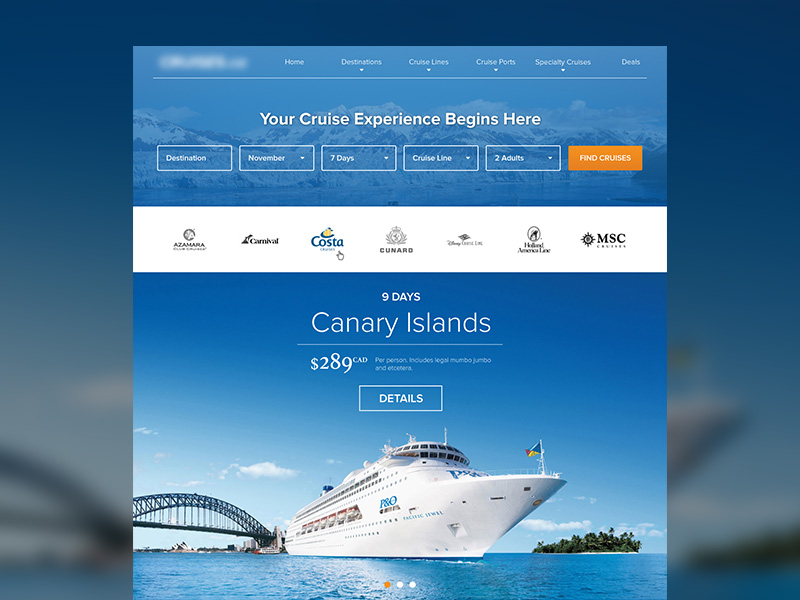The image showcases a travel-themed webpage with a blurry background for a refined focal point. The top section features a blue sky with snow-capped mountains and a lake, partially obscured to emphasize the central content. At the top, a navigation bar displays tabs labeled "Home," "Destination," "Cruise Lines," "Cruise Ports," "Specialty Cruises," and "Deals" on the top right.

Centered on the page, a prominent white text reads "Your Cruise Experience Begins Here." Below this, there are input fields for selecting a destination, a date in November, a 7-day duration, a cruise line type, and specifying 2 adults. An orange "Find Cruises" button is positioned on the right side.

Just beneath, logos of sponsors include MSC, Cunard, Costa, and Azamara flanked by a promotional offer: "9 days, Canary Islands, $289 CAD per person" along with a "Details" button.

A white P&O cruise ship elegantly sails in the lower segment, with a lush green island to its right. A blue-toned bridge and ocean complement the idyllic scene, all set against the same atmospheric background, albeit blurred to maintain focus on the central content.